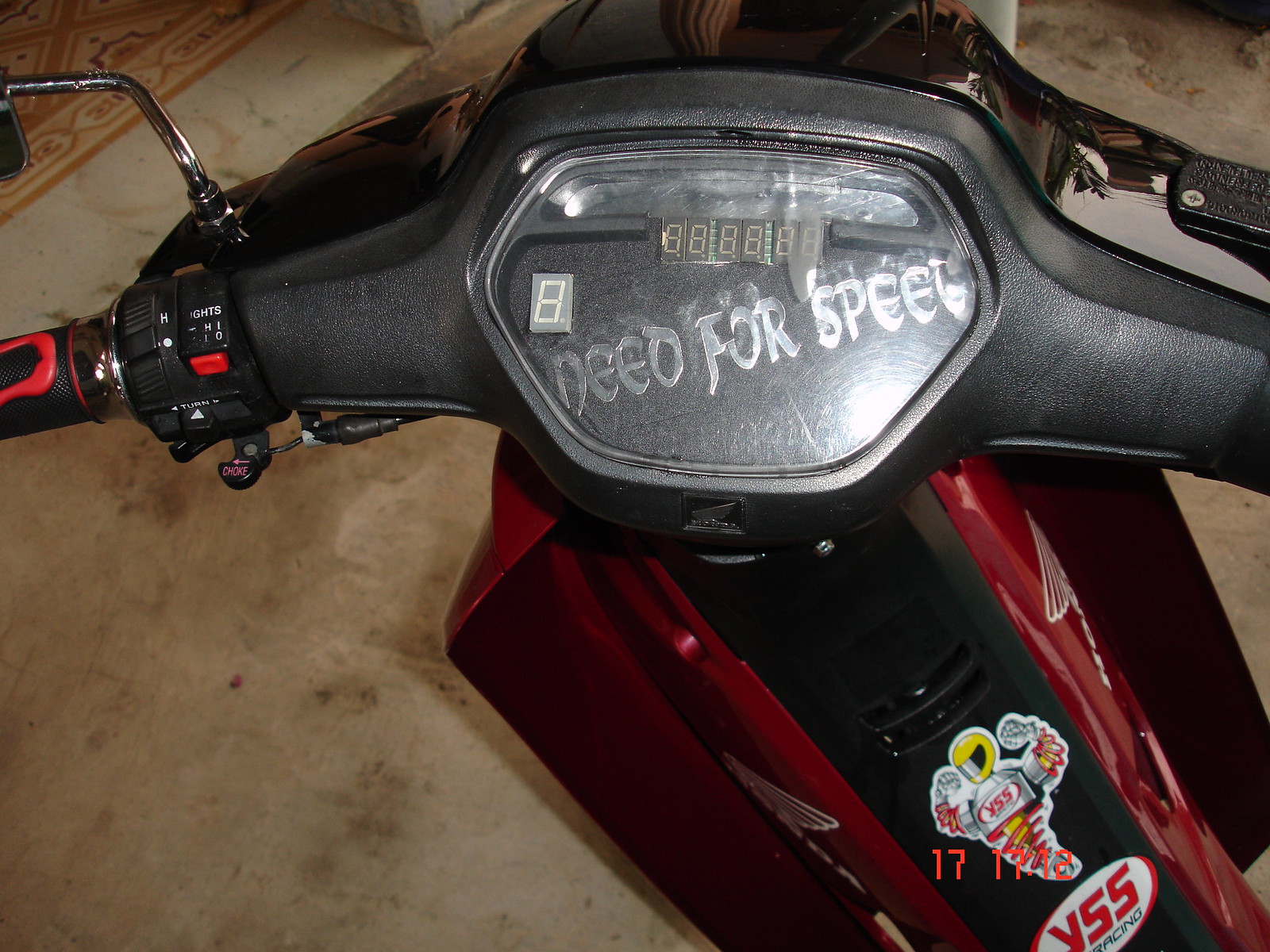This photograph captures the front section of a sleek motorcycle. The focus is on the handlebar area and the front body of the bike. The centerpiece of the handlebars features a clear plastic gauge displaying a series of numbers: '8888888' with an additional '8' to the left. Intriguingly, the phrase "Need for Speed" is emblazoned across the gauge. The handlebars themselves extend outward in a striking combination of black with red accents. Beneath the handlebars, the motorcycle's body showcases a bold red and black color scheme. Notably, a distinctive decal adorns the middle section, accompanied by another decal below it that reads 'VSS'. The background reveals the concrete floor of a garage, adding a gritty, industrial context to the image.